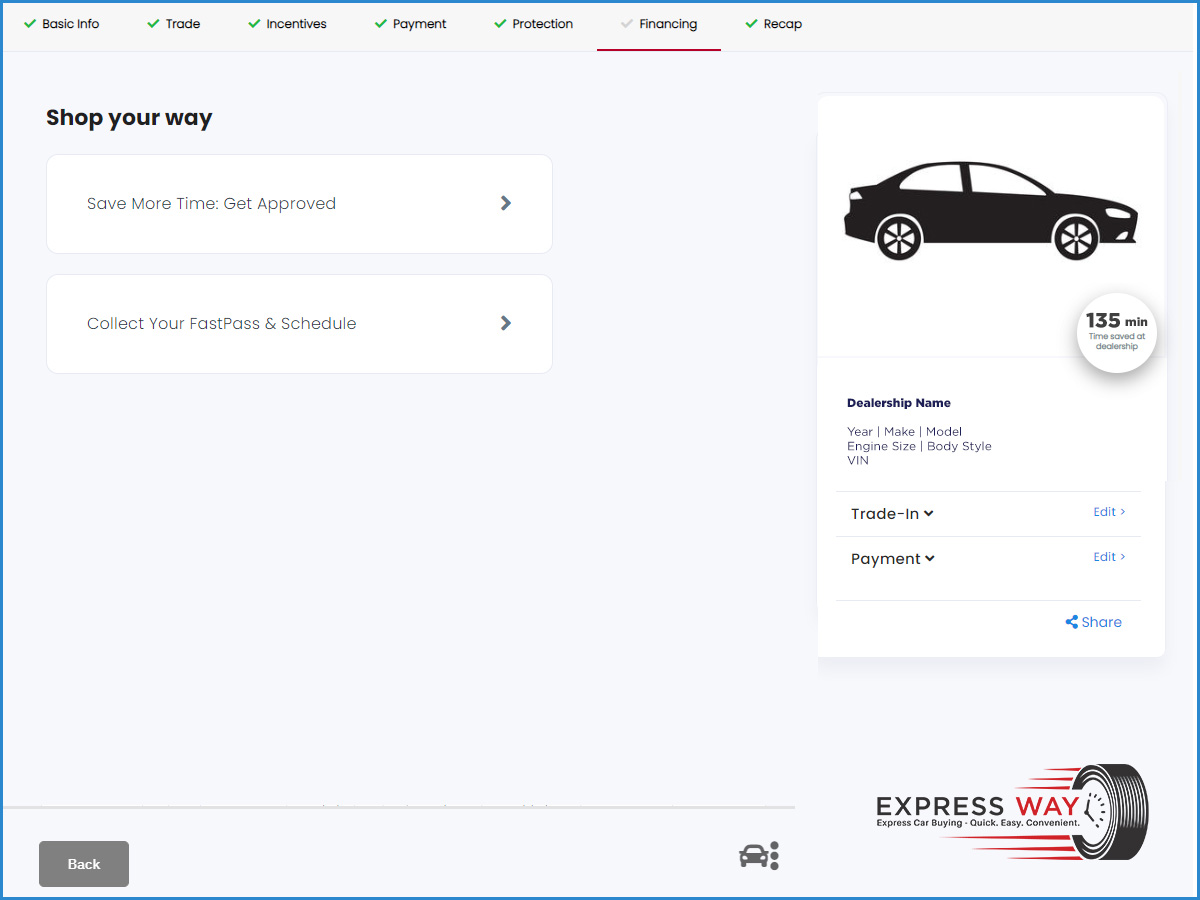Screenshot of a car purchasing app called Expressway, featuring their logo with the tagline "Express Car Buying - Quick, Easy, and Convenient". Displaying the "Shop Your Way" menu, it offers two key options: "Save More Time to Get Approved" and "Collect Your Fast Pass and Schedule". An illustration of a car is located to the right of the menu. Below the illustration, users can input details such as dealership name, year, make, model, engine size, body style, and VIN. There's also a scroll-down option for trade-in details and another for payment choices, allowing users to specify their search criteria.